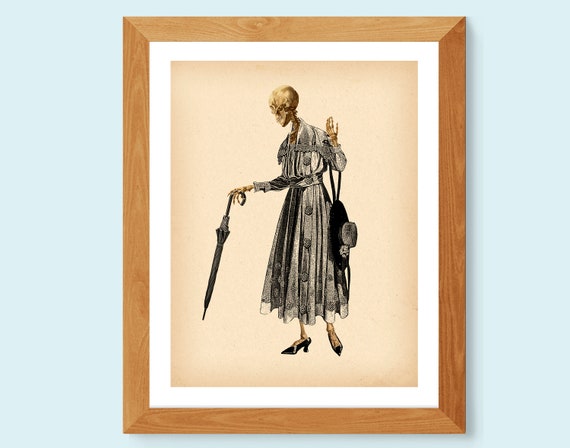The image is set against a light blue background and showcases a painting encased in a dark brown frame, which includes an inner white border that frames the artwork itself. The painting features a tan background and depicts a full skeleton, dressed in a long-sleeved, black and gray dress adorned with a vertical floral pattern. The skeleton's head is turned slightly to the side, revealing the bony details of its skull. It holds a closed, curved-handled umbrella in its right hand, while its left elbow supports a black, wide-brimmed hat tied with a ribbon. Black high heels are on its skeletal feet, emphasizing a fashionable, albeit macabre, appearance.